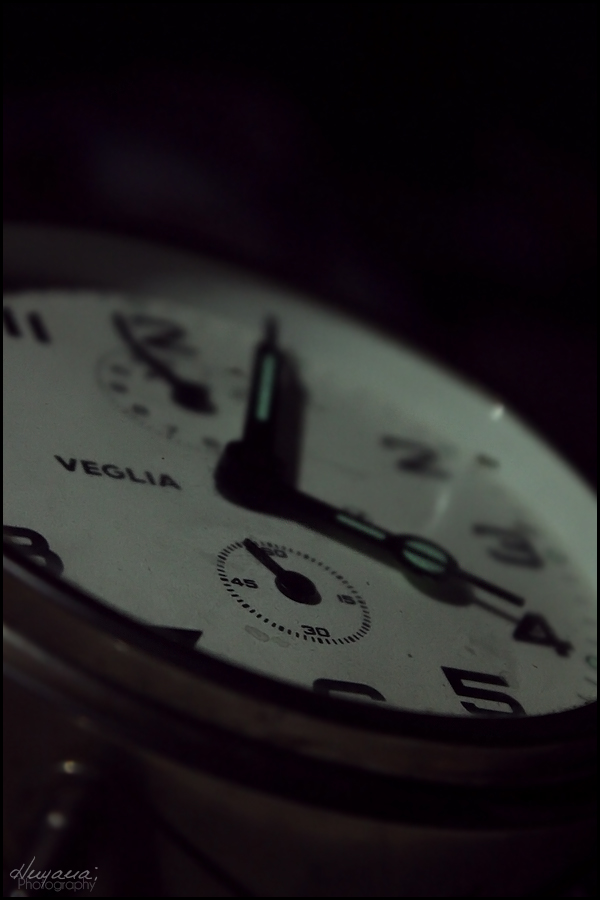This image features a detailed close-up of a wristwatch face, prominently displaying the brand name "VEGLIA" in black capital letters on the middle left. The watch has a white, circular face with large black numerals indicating the hours. The hands of the clock are black with a strip of green glow-in-the-dark coloring, appearing robust and wide, except for the thin black second hand. The time shown is just after 4 o'clock. There are two additional smaller dials, situated at the upper and lower portions of the main face, possibly for different time zones, each with very small black hands. The watch face is leaning slightly upward and is encased in what appears to be brass metal. The background of the image is very dark, nearly black, accentuating the watch face. In the left-hand corner, below the VEGLIA name, is an additional small signature written in white ink, which is difficult to read but seems to spell H-U-Y-A-U-A. Additionally, there are two small dots beneath this signature. The image is taken at a diagonal angle, focusing solely on the watch face.